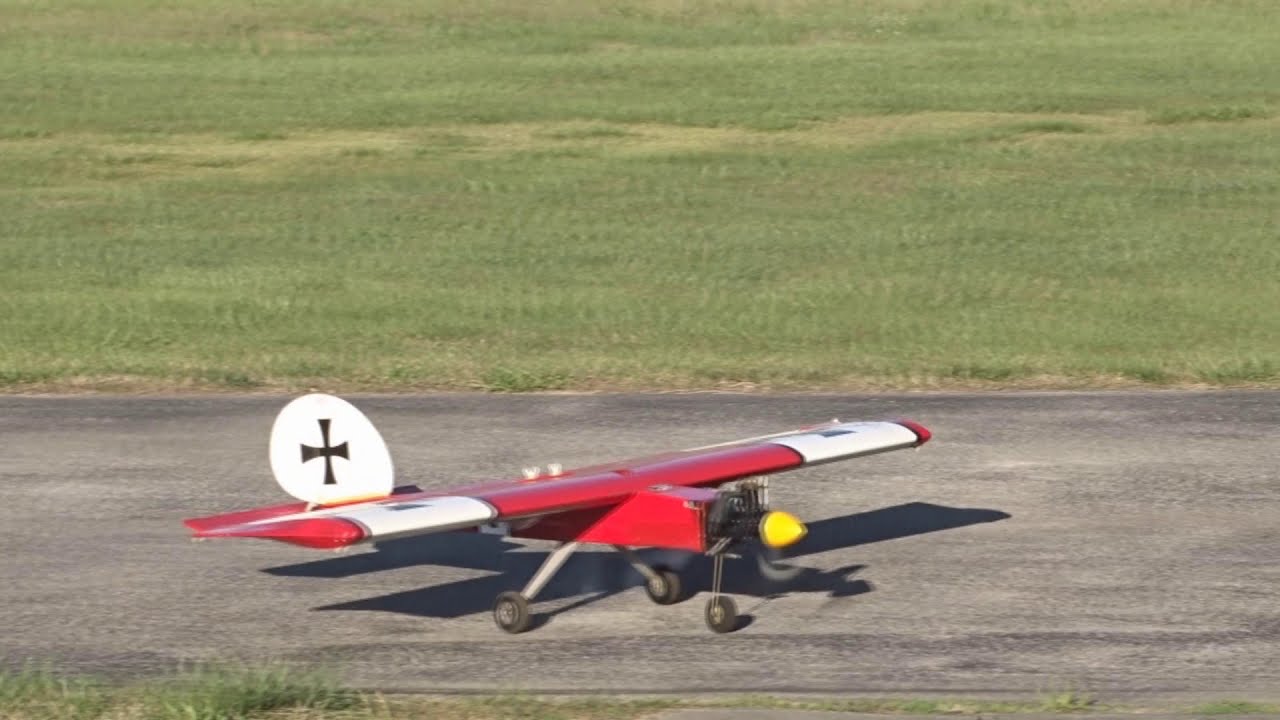The photograph depicts a model airplane reminiscent of a German World War I or II aircraft resting on a gray cement runway. The plane features a predominantly red body and wings, with white wing tips and white blocks at the end of each wing, each adorned with a cross design. The nose of the plane is painted yellow and extends into a white propeller with a black cross at its center. The runway is situated in a rural area, having the appearance of an airstrip rather than a conventional airport, and is bordered by a grassy field. There are no trees, and the shadow underneath the plane suggests the sunlight is coming from behind it. The overall scene exudes a nostalgic air, emphasizing the intricate details of the model airplane and its vintage aesthetic.